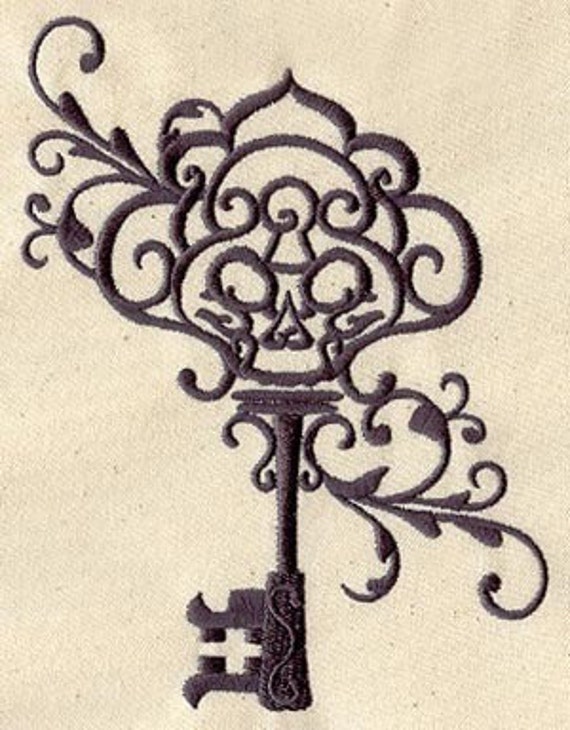This photograph showcases an intricate embroidered design on an uncolored, unbleached, light tan fabric, which has a diagonal texture and a thick appearance that suggests a vintage or antique quality. The embroidery is done in dark brown thread, not quite black, and appears to be machine-stitched. The design features a highly elaborate, old-fashioned key pointing upwards, with the part intended to go into the lock facing downward to the left. The key is richly decorated with swirling tendrils and leaf-like embellishments reminiscent of Indian designs, looping around the key in a detailed scroll pattern. Notably, the top of the key features an ornate skull, with a keyhole positioned between its eyes and a notable gap where the teeth would be. The "bit" or "blade" of the key, located at the bottom, consists of a cross shape, adding to the intricate and antique aesthetic of the overall design.